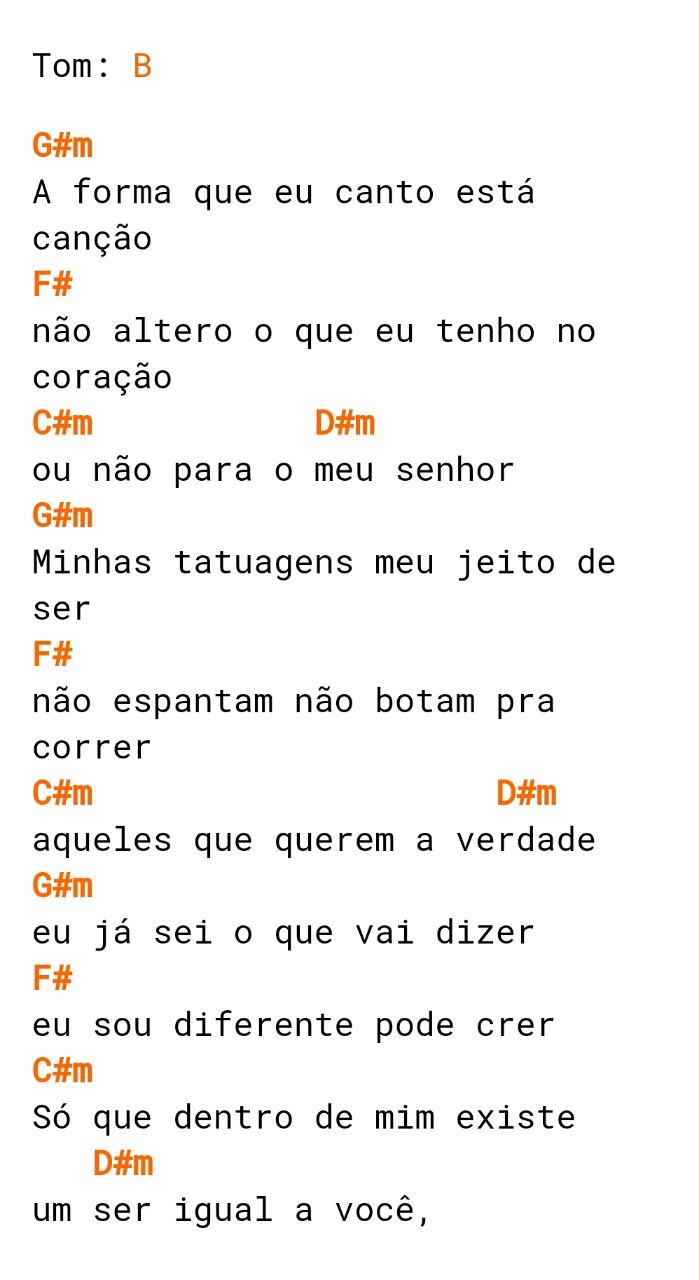The image appears to depict a script formatted in a vertical arrangement, with lines of text alternating in black and orange colors. At the top, the black text reads: "Tom:" followed by an uppercase orange "B." Below that, an orange "G#M" is present. The next line, in black, says: "a forma que u canto esta," followed by "concao" in black. Subsequently, an orange "F#" is visible, followed by the black text: "now altero o que tenho no," and then "coracao." This pattern continues with alternating orange and black text, showcasing a mix of musical notes and lyrics. The orange text includes musical notations like "C#M," "D#M," "F#," and "G#M," interspersed with black text such as "o nao paro o meu senhor" and "Minas tatucuens meu jeito desier." Further down, "nao espantam nao potam pracorer" and "quellas que querem e verdade," in black text, are paired with orange musical notes. It concludes with lines like "yo sou diferente para crer" and "um ser igual a vos" in black, maintaining the consistent alternating pattern of orange and black text throughout.